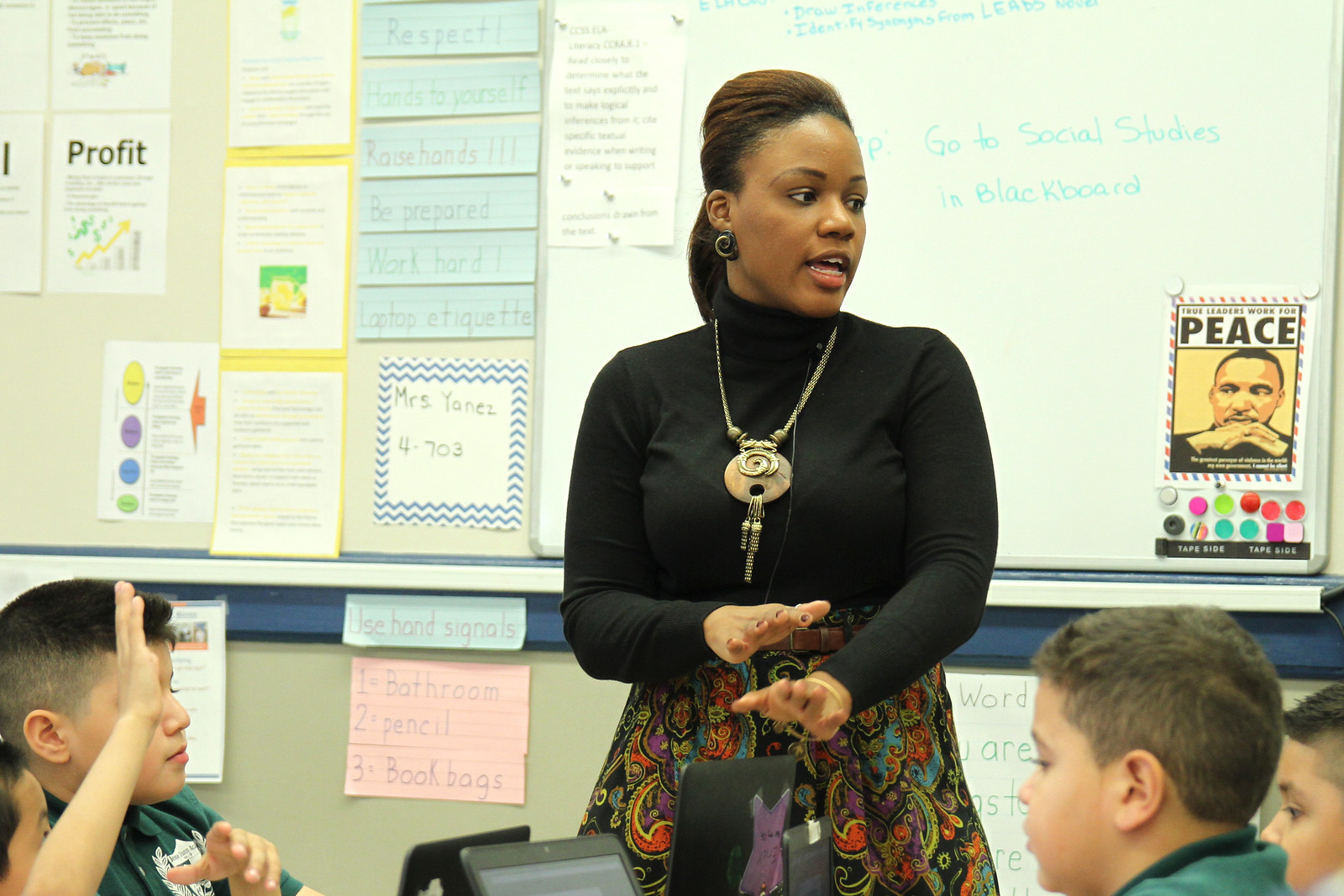In the classroom image, an African-American female teacher stands at the center, facing slightly to the right and making expressive motions with her hands. She is elegantly dressed in a long-sleeved black crewneck shirt paired with a floral print dress that features colorful spirals in shades of red, yellow, and purple. Around her neck, she wears a striking golden-hued necklace with an artifact-like design, including a circle with a pendant hanging from it.

Behind the teacher, a whiteboard displays multiple handwritten notes in blue marker. Near the top, small, legible lines are visible, while the center prominently reads, "Go to Social Studies in Blackboard." The bottom right corner of the whiteboard showcases a poster with the word "Peace" in black letters above an image of Martin Luther King Jr. looking slightly to the left. Below the poster, two rows of round magnets can be seen. To the far left of the whiteboard, a bulletin board is filled with various pinned flyers and papers, some of which seem to include lesson plans and classroom rules written in children's handwriting with phrases like "respect," "raise hands," and "be prepared."

In the foreground, four children with short hair, mostly boys wearing green shirts, are visible along the edges of the image. One boy on the far left, identifiable by a white emblem resembling a shield with a wreath on his shirt, raises his hand to ask a question. The tops of other students' heads can be seen, suggesting their attentiveness to the teacher's lesson. Overall, the scene depicts an engaging and organized classroom environment.